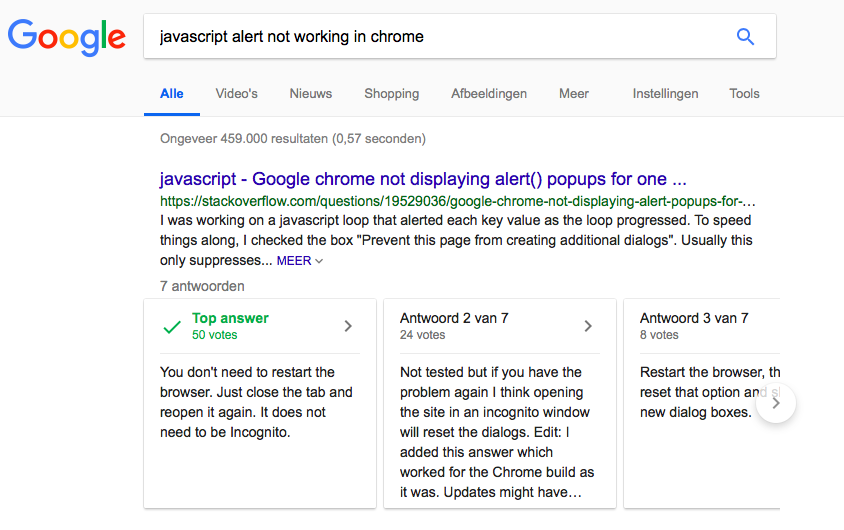This is a screenshot of a Google search results page. At the top, there is a light gray horizontal rectangle. On the left side of this rectangle, the word "Google" is displayed in the iconic multicolored Google logo. To the right of the logo, there is a rectangular search bar. Inside the search bar, the search query "JavaScript alert not working in Chrome" is written in bold black text. Further to the right, within the search bar, there is a blue magnifying glass icon.

Approximately three lines below the search bar, aligned horizontally, is a menu bar. The first menu item, "ALLE", is displayed in blue text and underlined in blue, indicating that it is the currently selected tab. To the right of "ALLE" are additional menu items written in gray text; these items are in a language that is not understood, totaling eight menu options across the bar.

Below the menu, the search returns are displayed. The first search result has a title in blue text: "JavaScript - Google Chrome not displaying alert (pop-ups)". The title is followed by an ellipsis, indicating that it is truncated. Underneath the title, there is a green hyperlink to the source article. Below the hyperlink, there are three lines of black text summarizing the content.

Further down, there are three white squares outlined with thin gray lines, each representing individual answers related to the search query. The first square is positioned on the left, the second in the middle, and the third on the right side of the screen. Each box likely contains additional information or solutions related to the query but are not detailed in the screenshot description.